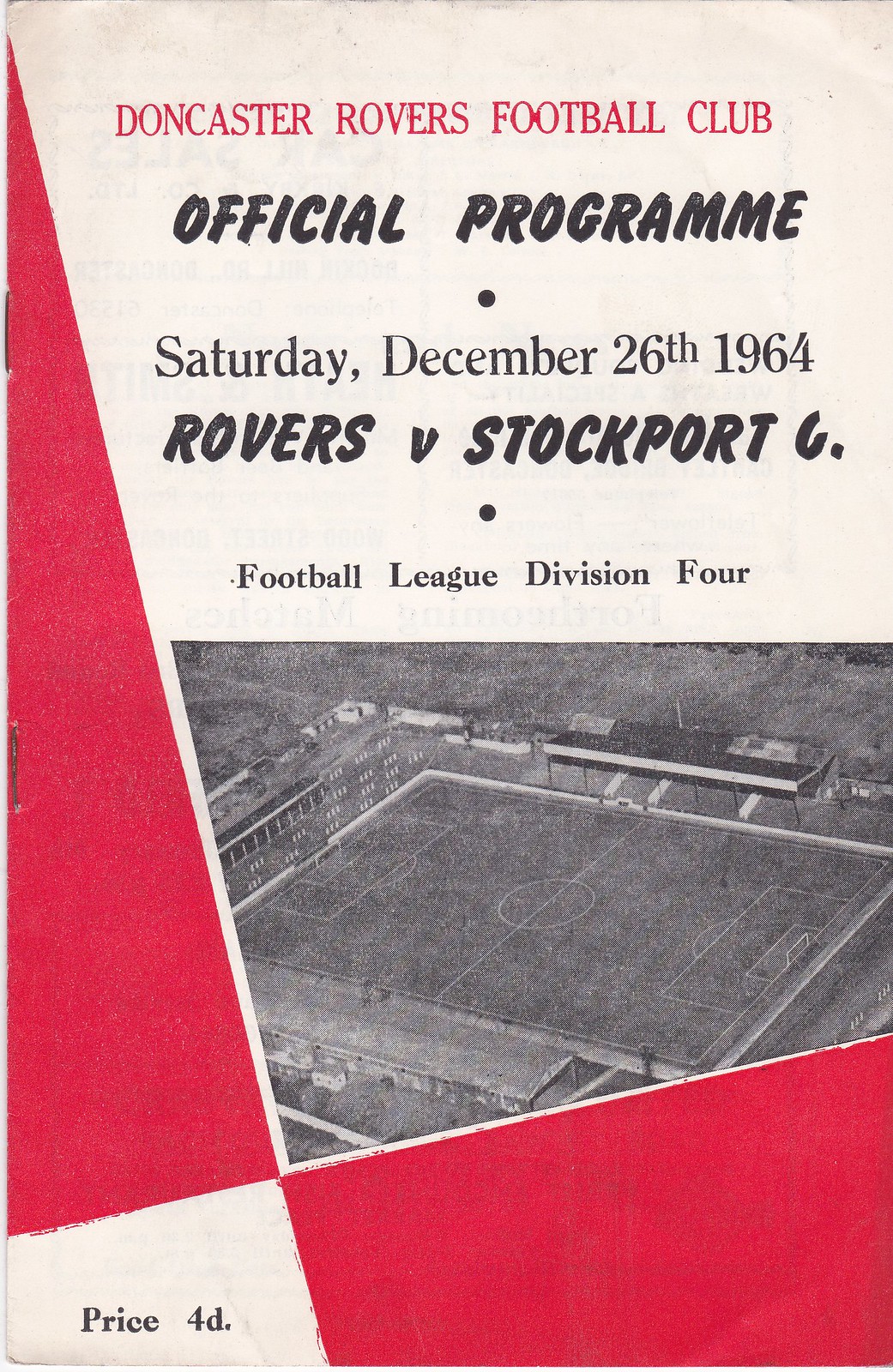The front cover of the magazine or sports game program has a predominantly white upper background with a beige tone underneath. A tall red rectangle runs along the left side, while a red parallelogram section occupies the bottom right corner. In the bottom left corner, there's a white rectangle housing black text that reads, "Price, 4D." 

At the center, the cover features a grainy, black-and-white aerial photograph of a soccer field, which appears empty. 

The top section of the cover boasts the title "Doncaster Rovers Football Club" in bold red capital letters. Below that, in black text, it reads, "Official Program," followed by "Saturday, December 26th, 1964," "Rovers v. Stockport C," and "Football League Division IV."